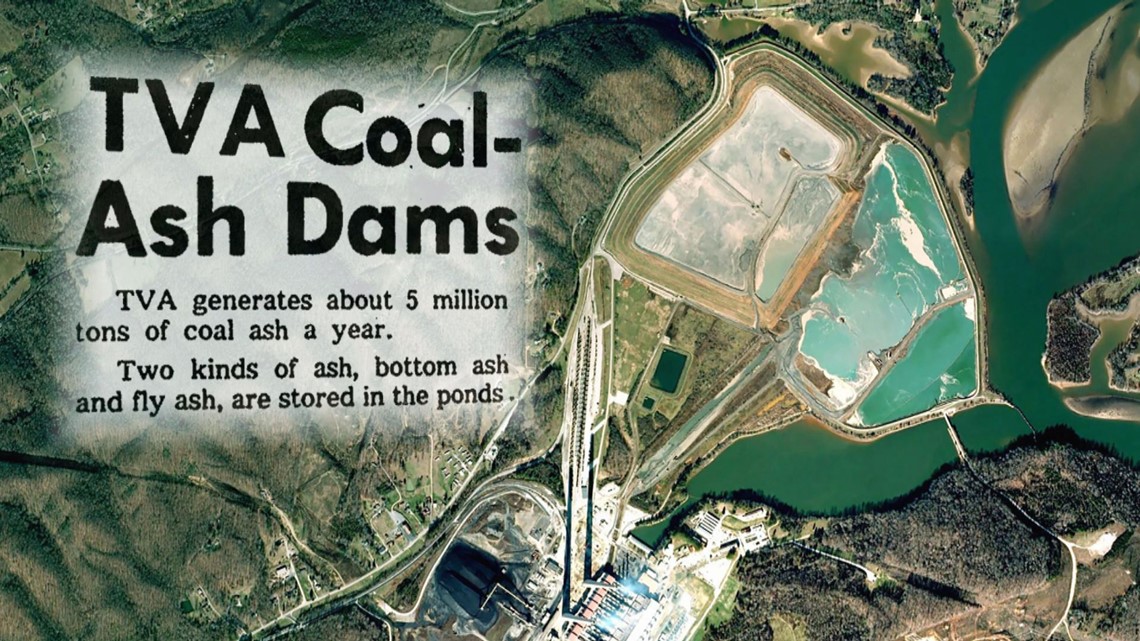The aerial image depicts a TVA coal ash dam surrounded by sprawling land and trees, devoid of residential areas. The central feature is a sprawling body of water exhibiting multiple hues: a dark green stream flowing into the dam transitions into a lighter green, almost pretty water held in by the structure. The water in some backup portions of the dam appears whitish and sandy. Two ponds for storing coal ash, specifically bottom ash and fly ash, can be seen within the landscape. The text overlay, situated towards the left on a faint white background, is in dark black print and reads: "TVA coal ash dams" followed by "TVA generates about 5 million tons of coal ash a year. Two kinds of ash, bottom ash and fly ash are stored in the ponds." Additionally, the image shows the coal plant that controls the dam, alongside some roads and darkened areas attributed to coal activity. The image also features a combination of tealy-aqua green water transitioning into lighter bluish tones, adding to the visual appeal of the landscape.